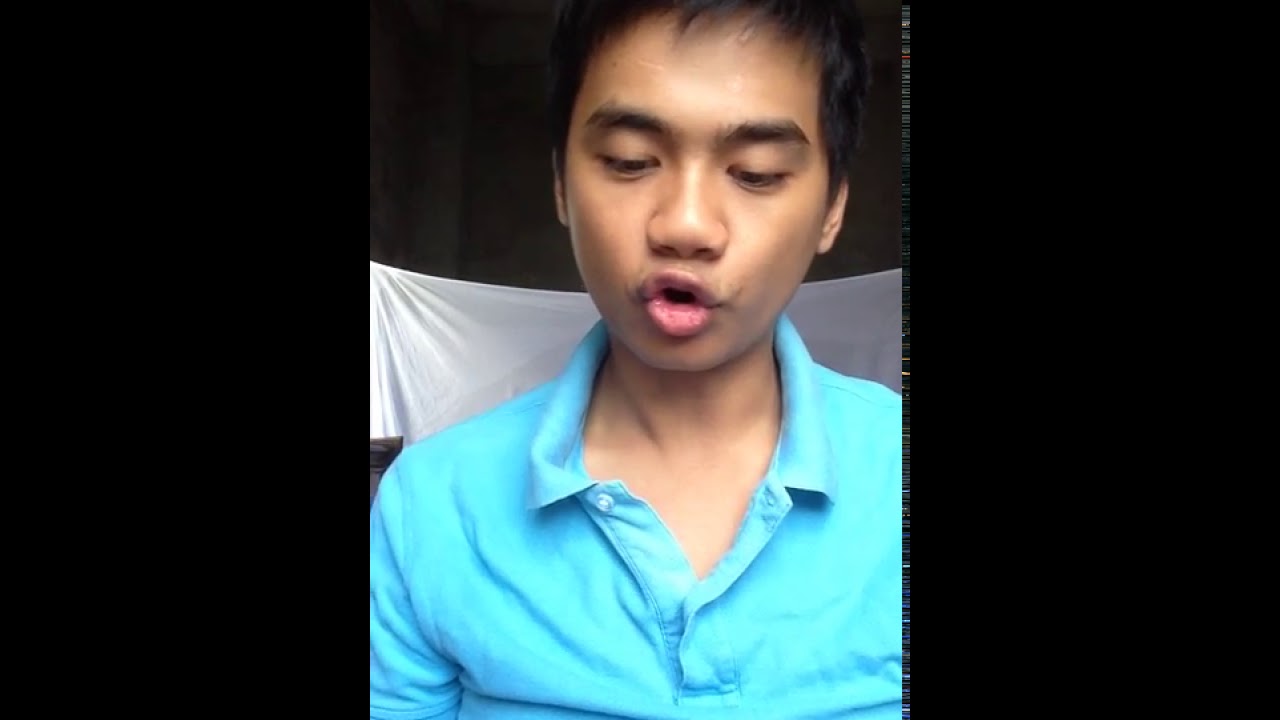In the image, there's a young Asian man, likely in his early 20s, who is the main focus. He is captured from mid-chest up, with the top of his head cut off by the frame, highlighting his straight, combed-down short black hair, high forehead, and dark black eyebrows. His eyes, featuring heavy monolid eyelids, are looking downward, revealing glimpses of his dark brown or black eyes. The man's broad, flat nose and lips forming an O shape suggest he might be about to sing, whistle, or speak. He is dressed in a light blue collared polo shirt with the top button undone. Behind him, there's a white sheet hanging horizontally from just below his shoulders to his cheekbones, with a black background above. The image is framed with thick black borders on the left and right sides, making the central portion of the image taller than wide, giving the impression that he might be engaging in a video or live stream on social media, potentially on platforms like TikTok, YouTube, Instagram, or Twitch.